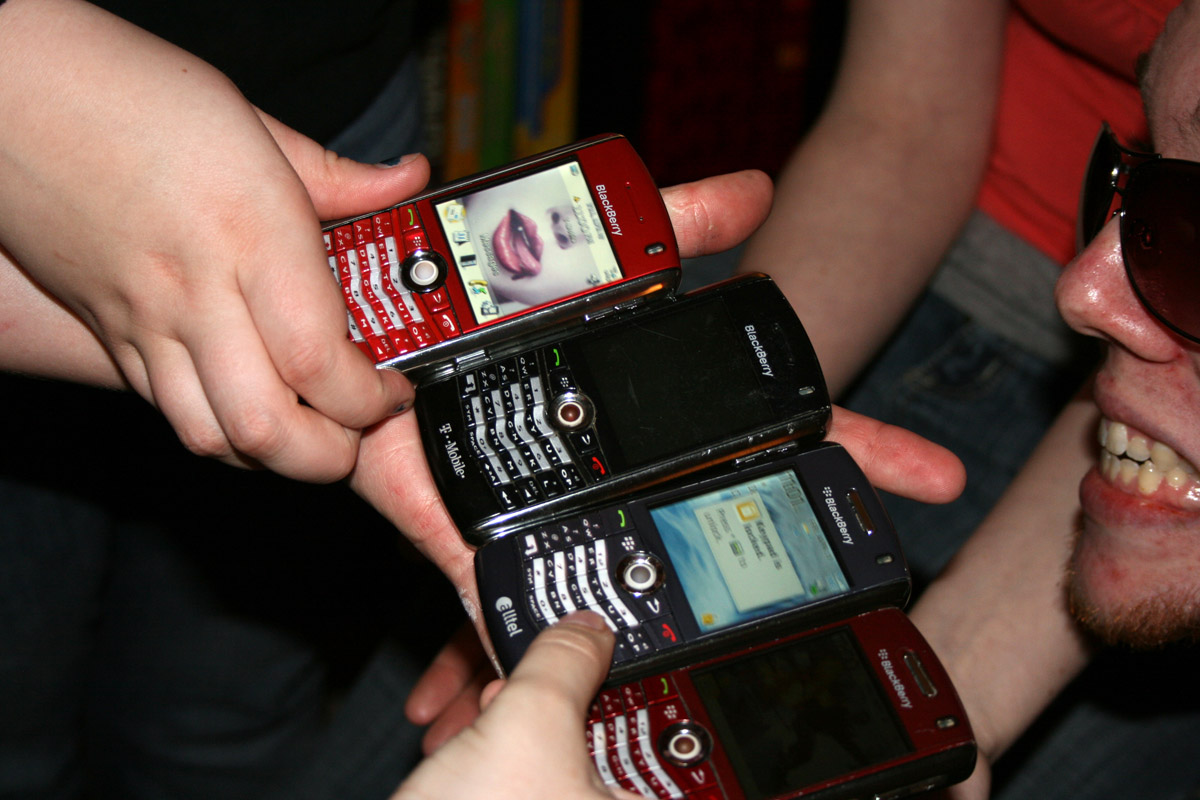This vibrant, close-up image captures a nostalgic moment where a group of friends showcase their cherished BlackBerry smartphones. Central to the photo are four distinct BlackBerry phones held by several hands, which vary in skin tone and share a reddish tint on the fingers. The arrangement starts at the bottom with a deep red BlackBerry that features white keys and a display showing a woman's face with red lipstick and her tongue sticking out. Above it lies a black BlackBerry with white keys, its screen displaying a blue notification with the time set at 11:01. The next phone, colored steel blue, contrasts with its gray keys and an inactive display. The final phone at the top, in a bright red hue, also showcases white keys and another angle of the woman's face with red lipstick. Off to the right, a man with a goatee and sunglasses smiles widely, showing slightly yellowed teeth and acne. The background fades into an indistinct mix of blue jeans and shaded areas, ensuring the intricately detailed phones and the friendly exchange remain the focus of this vintage snapshot.